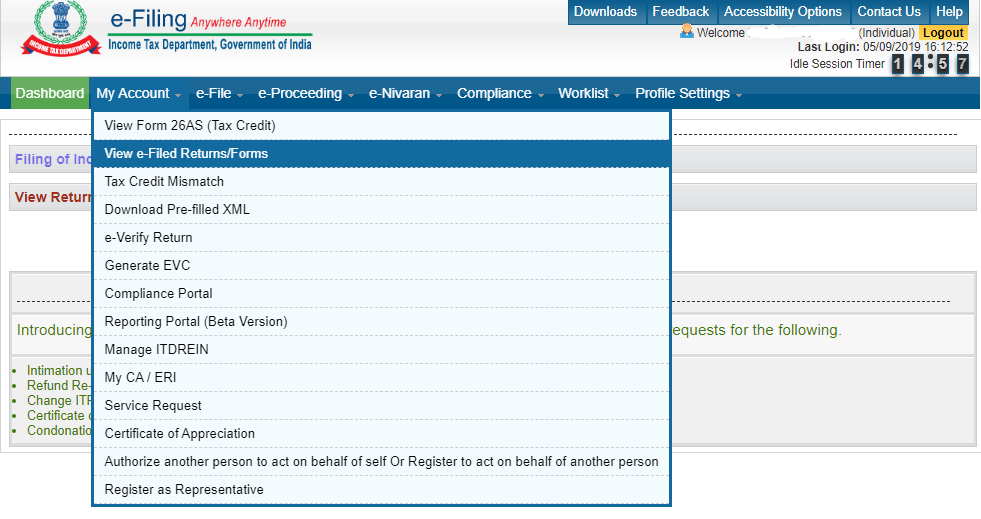This landscape photograph captures the homepage of the Income Tax Department of India's e-filing portal. At the top, a gray header features an icon on the left containing a green hollow circle with a blue object inside, overlaid with a red curved banner and white lettering. To the right of the icon, the text reads "e-Filing" in blue and "Anytime Anywhere" in red. Further to the right, a horizontal green border bears the text "Income Tax Department, Government of India."

On the top right corner of the gray header, a blue menu offers options such as "Downloads," "Feedback," "Accessibility Options," "Contact Us," and "Help." Below the header, a greeting welcomes the user (name redacted) in white text, accompanied by a yellow "Logout" button.

Dominating the central part of the interface, the dashboard is marked by a green box with white lettering. Featured options on the dashboard include "My Account," "e-File," "e-Proceeding," "e-Nivaran," "Compliance," "Worklist," "Profile," and "Settings." The "My Account" section is selected, revealing a drop-down menu with a bluish-green background highlighted by "View Form 26AS" and "View e-Filed Returns," followed by other options in black text.

The bottom of the image contains green text within a gray-bordered area, merging seamlessly with the overall color scheme and layout of the e-filing portal's homepage. The website interface is well-organized, facilitating easy navigation and access to various functionalities.